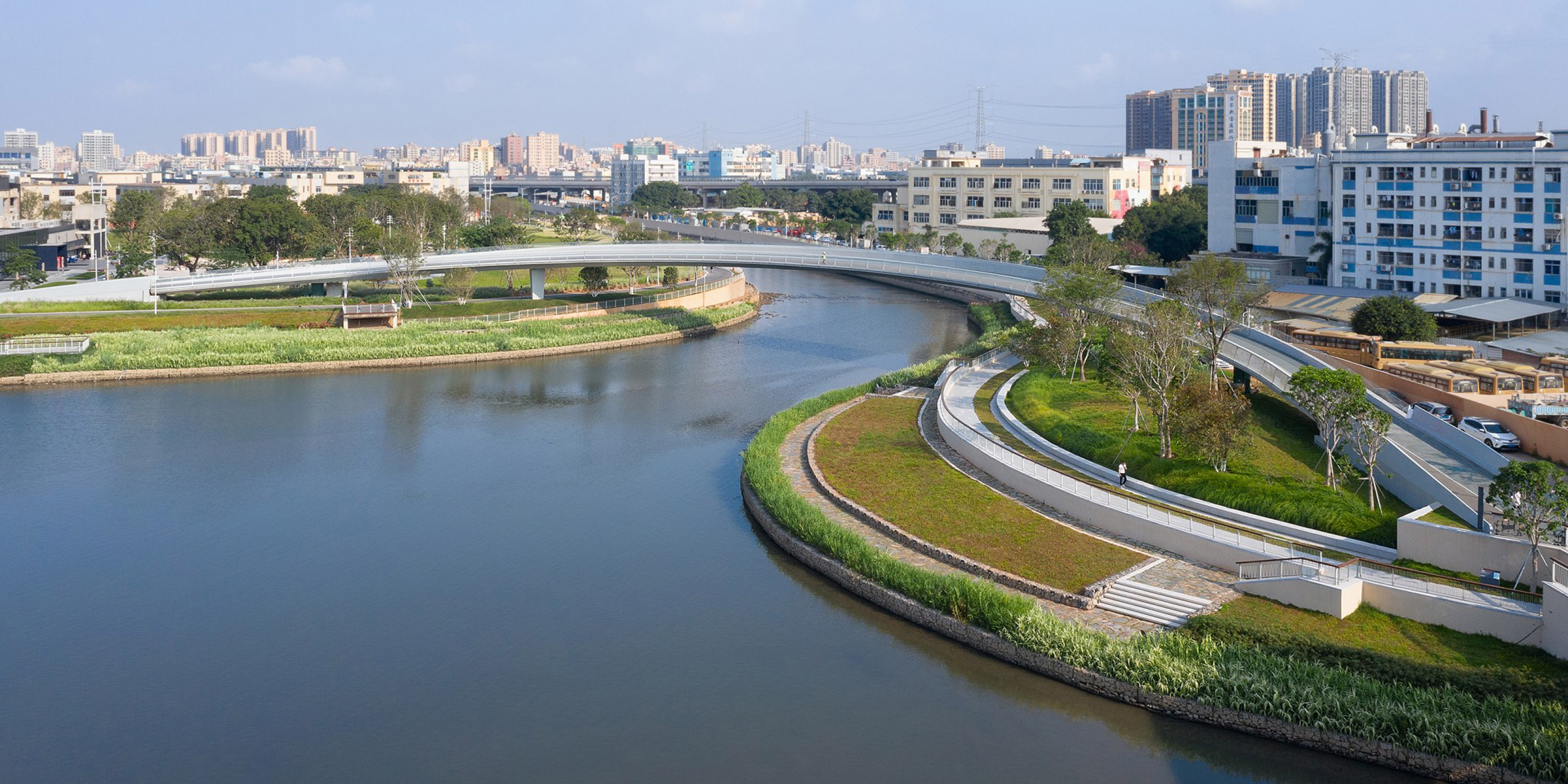The photograph captures a sprawling cityscape centered around a large, meandering river edged with neat greenery. Prominently visible is a bridge that spans the river, connecting the urban areas on either side. The buildings, predominantly industrial in appearance and painted in shades of white and grey, dominate the landscape. To the right, a cluster of yellow school buses can be seen in the background. The scene is bathed in bright sunlight under a light blue sky with very few clouds, creating a clear and vibrant atmosphere. The background features an array of tall buildings, including indistinct skyscrapers and apartment towers, underscoring the city's extensive scale. Additionally, there's a park where some people are seen walking, adding a touch of life and movement. Numerous cars populate the roads, and there is no visible text in the image. Hints of red accentuate an otherwise cool color palette dominated by blues, greens, whites, and grays.